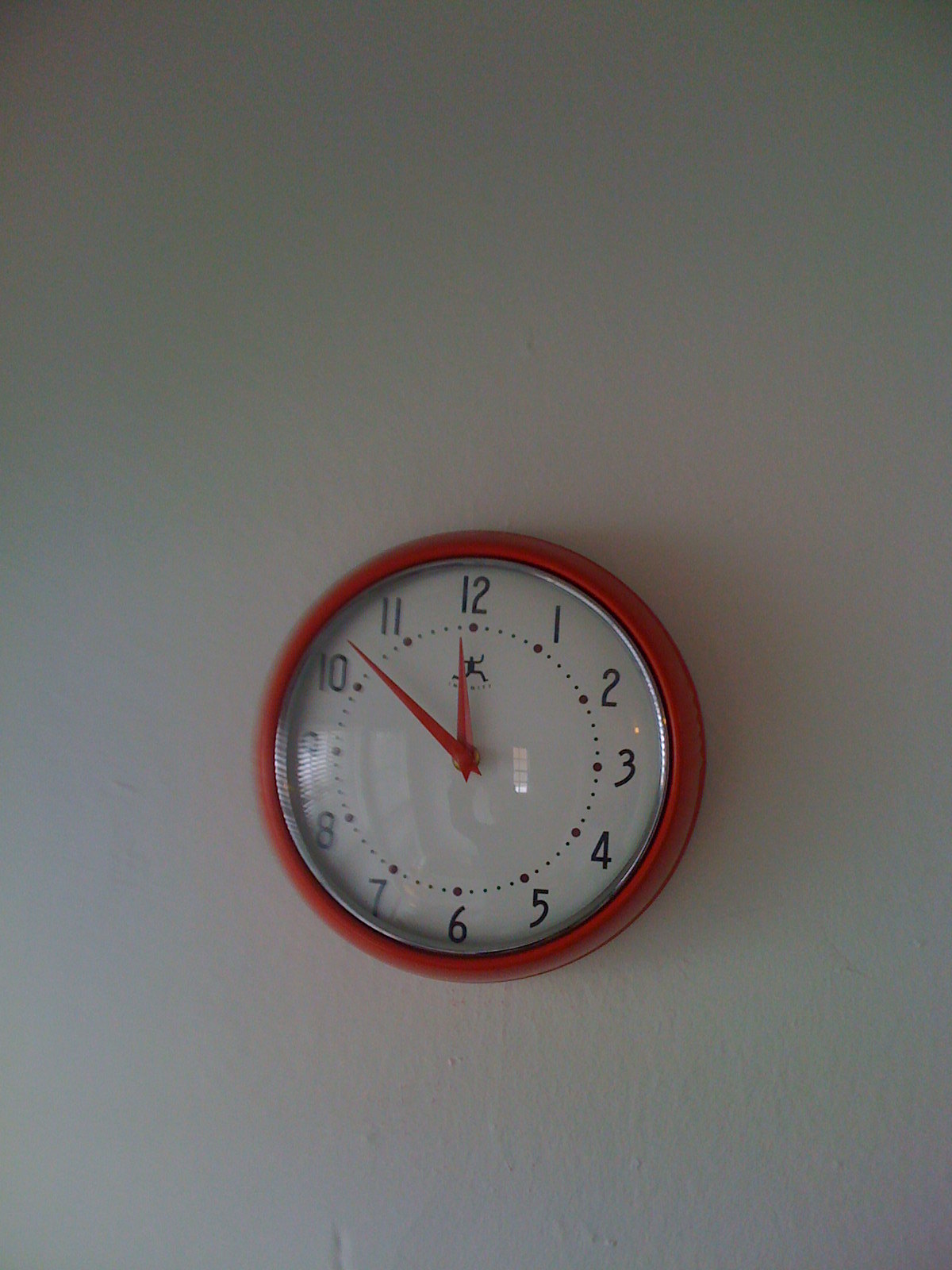This color photograph features a simple, clean composition showcasing a circular clock mounted on a white wall. The clock, positioned in the lower part of the image, has a bright red enamel casing and a glass front that is slightly reflective. The clock’s face is white with black numbers and red dots marking each numeral. The hands of the clock, which are also red, indicate the time is approximately 11:57. Notably, just beneath the 12, there is a small insignia of a stick figure running, although the accompanying text is not legible. A shadow, cast by the person taking the photo with a cell phone, falls across the clock, making it difficult to determine the photographer’s identity. The background reveals little about the setting, though faint reflections in the glass suggest the presence of Venetian blind-covered windows and possibly another window, hinting it could be in a living room or office. The room is well-lit, contributing to the clear and vivid appearance of the photo.